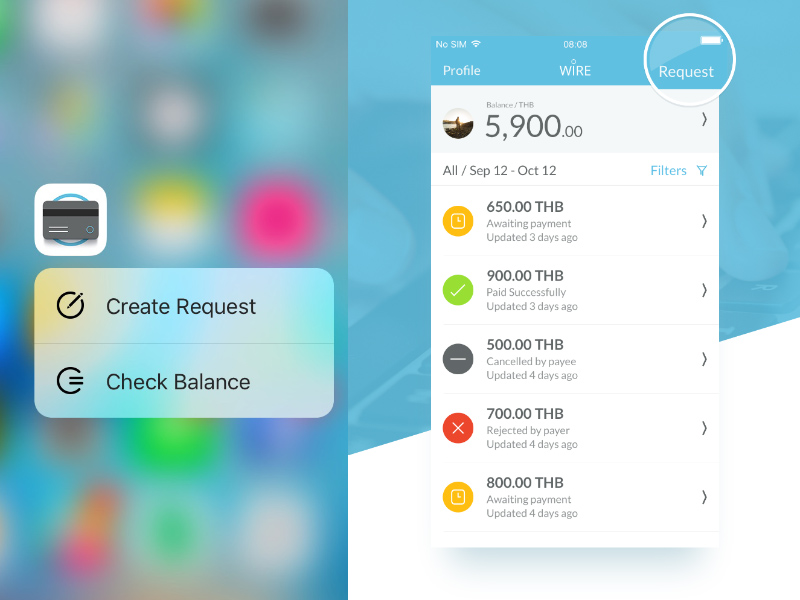**Description:**

The image is a screenshot featuring a split-screen interface with detailed financial transaction information.

**Left Half:**
- A long, rectangular blue box forms the background.
- Fuzzy, colored dots are visible, adding a soft texture.
- An inset white square displays the back of a credit card, rendered as an animated image.
- Below this, two options are presented:
  - "Create Request," represented by a pencil icon within a circle.
  - "Check Balance," featuring two lines on the right side of a circle.
  
**Right Half:**
- The top section displays various status indicators:
  - "No SM" for the Internet.
  - The time "08:08".
  - A full battery icon.
- A highlighted circle around the word "Request."
- Below this, there are three labeled options:
  - Profile
  - Wire
  - Request
- Underneath, there is a long, rectangular vertical box:
  - At the top, it says "Balance / THB".
  - A circle on the left contains an image of a lake with a person standing.
  - To the right of this image, the balance of "5,900.00 THB" is displayed, followed by a caret pointing right.
  - Below the balance, it states the date range "September 12 - October 12," with "All/September SEP" on the left and a blue "Filters" option with a corresponding icon on the right.
- Below this, a list of transaction updates is presented:
  - **First Item**: Orange circle, "650.00 THB awaiting payment," updated three days ago, with a caret pointing right.
  - **Second Item**: Green circle with a check mark, "900.00 THB paid successfully," updated three days ago, with a caret pointing right.
  - **Third Item**: Black circle with a minus sign, "500.00 THB canceled by payee," updated four days ago, with a caret pointing right.
  - **Fourth Item**: Red circle with an X, "700.00 THB rejected by payer," updated four days ago, with a caret pointing right.
  - **Fifth Item**: Yellow circle, "800.00 THB awaiting payment," updated four days ago, with a caret pointing right.

This detailed description meticulously captures the layout and content of the interface displayed in the screenshot, ensuring each element is clearly identified and described.